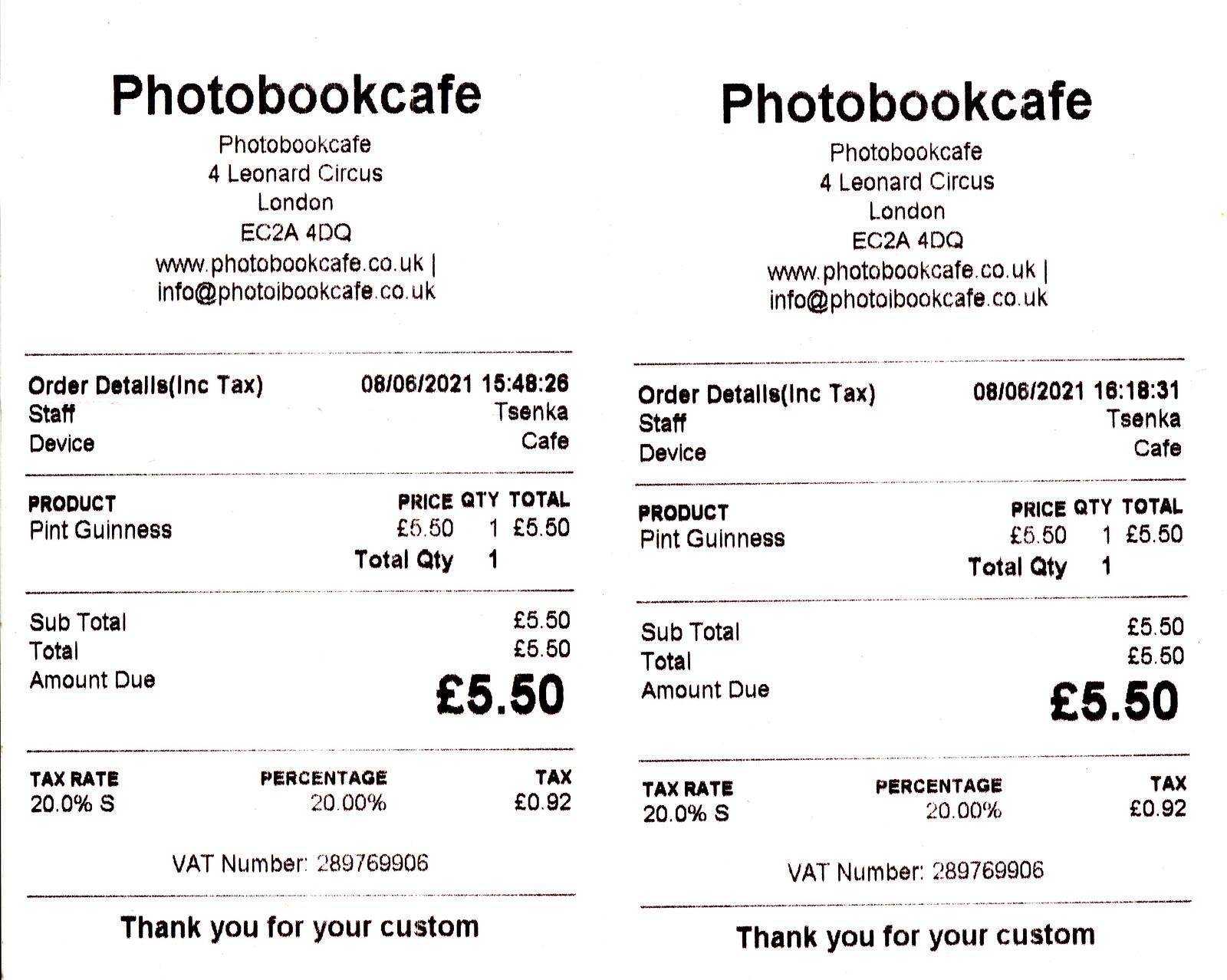This image showcases two side-by-side receipts from Photo Book Café, located at Poor Leonard Circus, London, EC2A 4DQ. Each receipt lists the website (www.photobookcafe.co.uk) and the email (info@photobookcafe.co.uk) at the top. Both receipts are for the same purchase of one pint of Guinness, priced at £5.50 each. The first receipt is timestamped August 6, 2021, 15:48:26, while the second one is timestamped August 6, 2021, 16:18:31. Both receipts show a 20% sales tax rate, with the total tax amounting to £0.92. The VAT number 289769906 is stated at the bottom of each receipt, just above the phrase "Thank you for your custom." The staff member listed on both receipts is Tecinska, and the device used for the transaction is labeled as 'caf.'